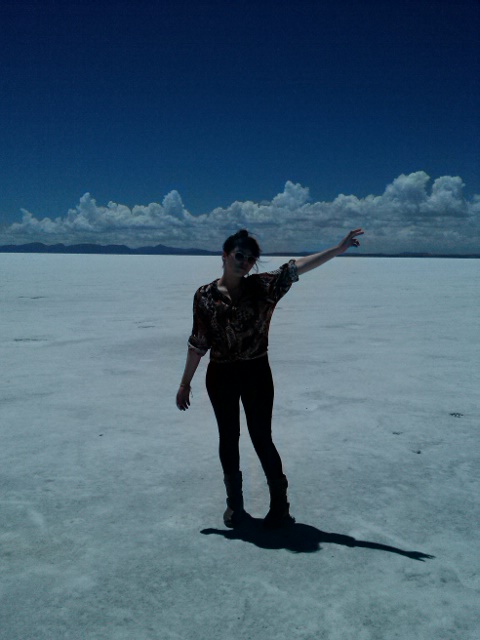In this evocative image, a young woman stands alone in what appears to be a vast, arid desert under a deep, dark blue sky. The scene is shrouded in darkness, lending an almost monochromatic feel to her attire, which consists of a darker-colored button-up blouse with rolled-up sleeves, dark tight pants, and tall boots. Her black hair is tied up, and she sports sunglasses that add to her enigmatic presence. She extends her left arm outward while her right arm rests by her side, adorned with a bracelet. Her shadow is clearly visible on the ground, which resembles a flat, whitish stone or concrete but is likely sand. Off in the distance, black mountains or hills can be seen under a horizon filled with numerous fluffy white clouds. A grayish filter seems to hang over the entire scene, enhancing the dramatic interplay of light and shadow across her figure.